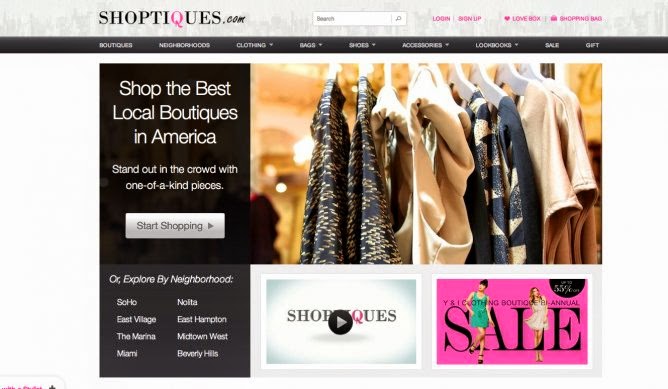Screenshot of the ShopTeeks.com website displayed on a desktop. At the top left, the ShopTeeks.com logo is prominently featured. The central top portion of the page contains a search bar, while the right side includes options for 'Login' and 'Sign Up.' Below this top navigation bar, there's a secondary menu with a darker gray background and white text. This menu provides links to various sections: Boutiques, Neighborhoods, Clothing, Bags, Shoes, Accessories, Lookbooks, Sale, and Gift.

On the left side, there's an inviting header that reads, "Shop the Best Local Boutiques in America. Stand out in the crowd with one-of-a-kind pieces." Below this header, a shiny silver button labeled "Start Shopping" encourages users to begin exploring the site. Underneath this call to action, the text "Explore by Neighborhood" introduces a section featuring eight wealthy neighborhoods.

To the right of this text, there is a generic image displaying high-end clothing on a rack, indicative of the website's focus on boutique fashion. Further down the page, the left side hosts a video, while the right side features a prominent ad for an ongoing sale.